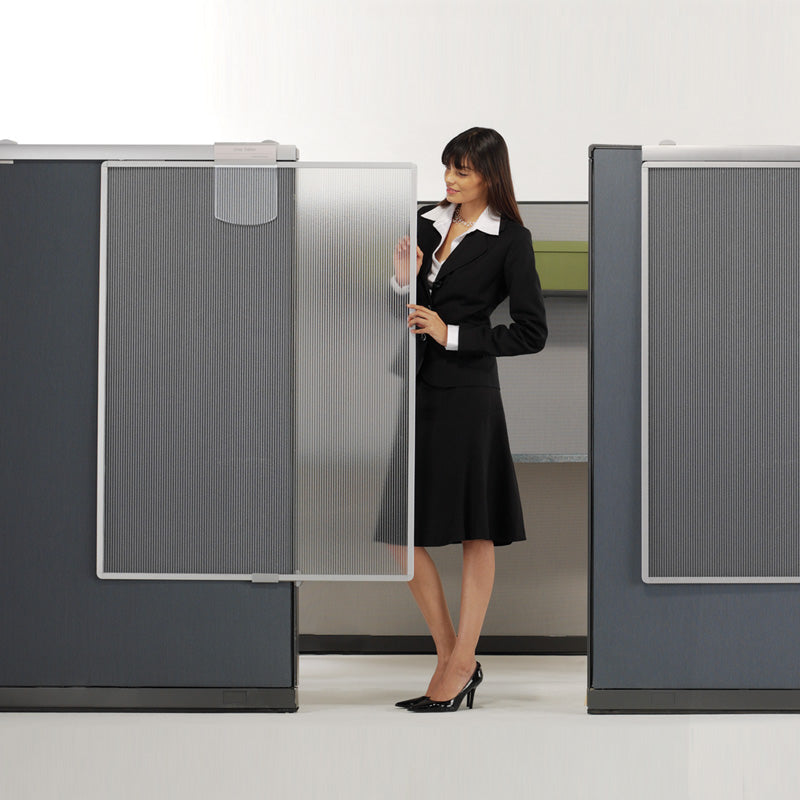A young woman, dressed in a classic black work skirt suit paired with a white button-down shirt and shiny black high heels, stands between two gray-felted, five-foot-high cubicle dividers. She has long, dark hair with bangs cascading to her shoulders. The woman is sliding a unique, new plexiglass door feature that acts as a privacy screen for the cubicle entrance. This innovative sliding door blurs the view, offering privacy while allowing some visibility, unlike a solid screen or curtain. Behind her, a cubicle wall features a green basket, hinting at the personalized touches within the office space. The woman gazes at the door intently, seemingly demonstrating its function and potential utility in the office setting.